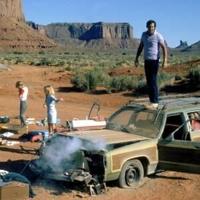In this small, square photograph set in a desert landscape, we see a scene reminiscent of a moment from the National Lampoon's Vacation movie. The image captures a stalled car, likely an old Jeep or station wagon, positioned towards the right side of the picture. The vehicle's worn beige hood is slightly ajar, emitting steam, indicating an overheated engine. The right-front tire is visibly flat, and miscellaneous items from the car are scattered around, suggesting a distressful situation. 

A man, recognized as the character played by Chevy Chase, is standing on the car's roof, dressed in a white T-shirt and dark pants, peering down at the steaming engine. Both the driver's and passenger's doors are open, hinting at recent activity or attempts to diagnose the car's issues. 

To the left of the car, two individuals, including a blonde woman in a long light blue dress, stand near the smoking hood. The woman, possibly the teenage daughter, points towards the car, her gesture clustering with concern and urgency. The backdrop showcases flat-topped plateaus and rocky escarpments, likely in Colorado, enhancing the sense of an isolated and challenging environment. The scene vividly portrays a family stranded in the desert, echoing themes of mishaps and journeys found in the classic comedy film.